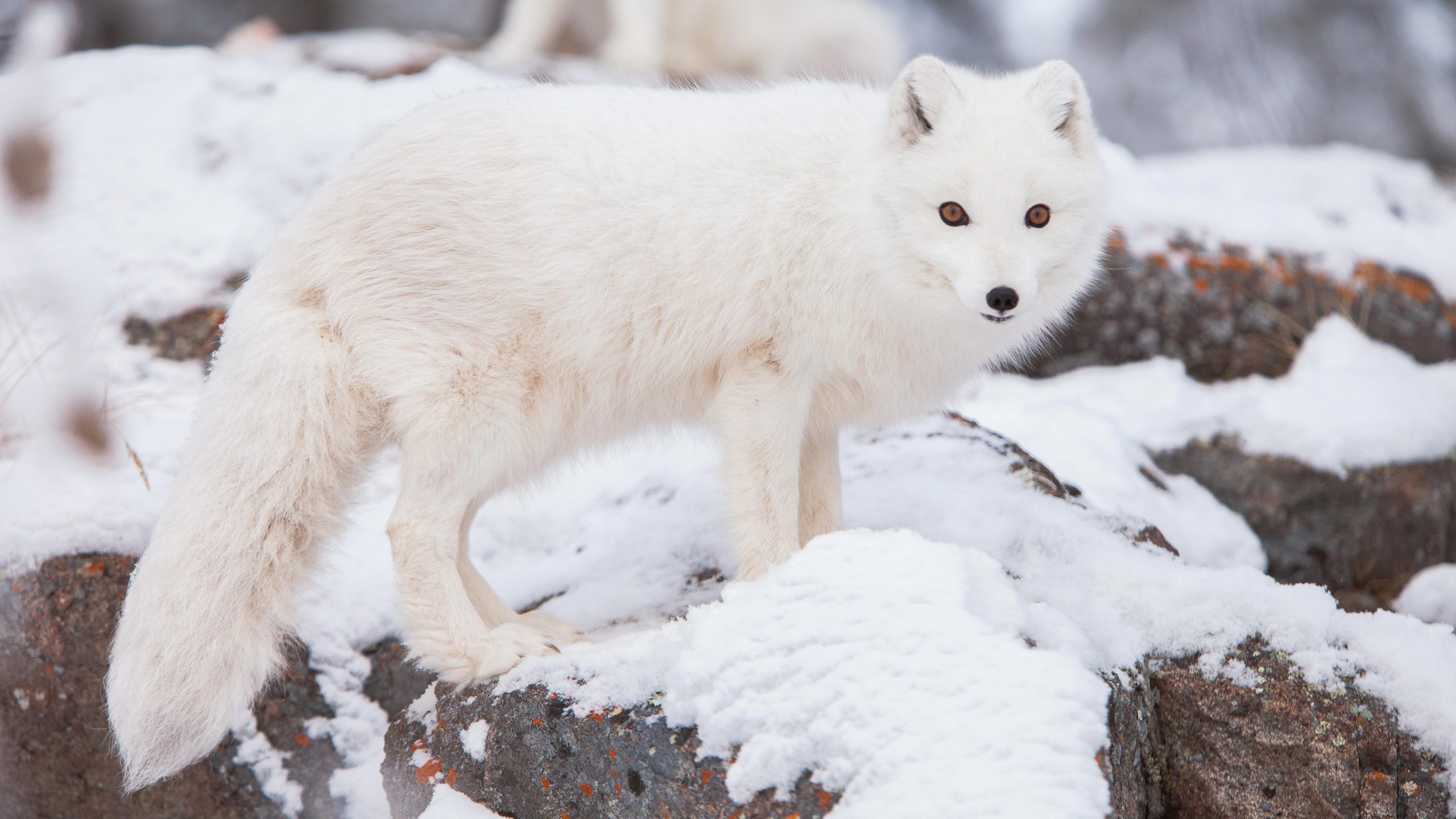The photograph depicts a medium-sized white wolf or arctic fox, distinguished by its thick, fluffy fur and striking yellow eyes outlined in black, giving it an eyeliner effect. The animal's small black ears, black nose, and black lips contrast against its predominantly white coat. It stands confidently on a formation of rocks, which are partly covered in white snow. The rocks beneath the snow display hues of gray and brown with occasional orange specks, possibly moss. The creature, positioned side-on but gazing directly into the camera, reveals its long, bushy tail and all four legs. The snowy landscape around it is slightly out of focus, emphasizing the animal as the central subject of this daytime outdoor photograph. The overall setting highlights the animal's natural camouflage within its wintry environment.